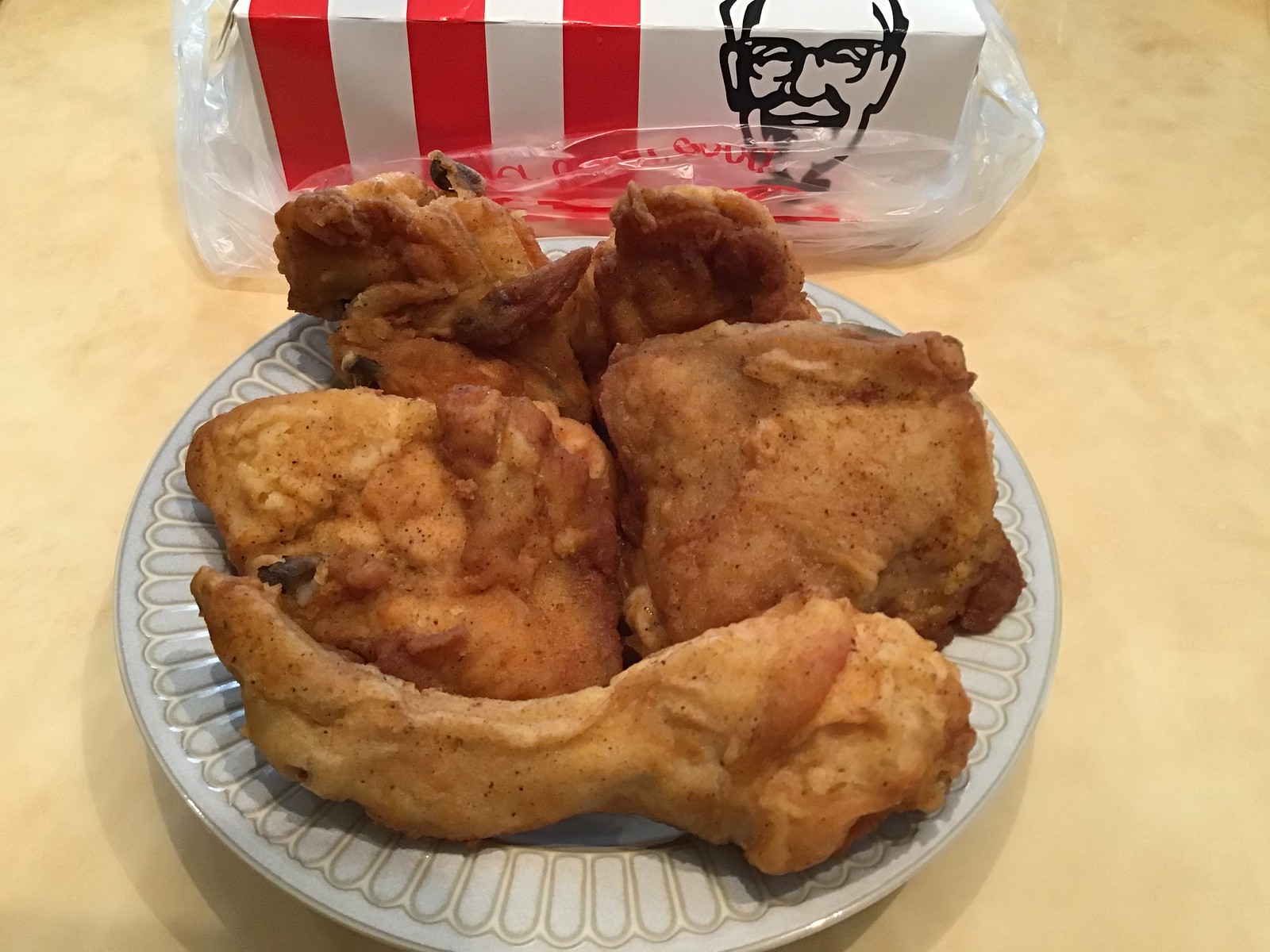A light tan table serves as the backdrop for a mouthwatering plate of fried chicken. The ceramic white plate, featuring petal-shaped detailing along the rim, holds six pieces of golden-brown KFC chicken in varying sizes and shapes, including drumsticks and thighs. Behind the plate, a KFC box is partly visible, marked by three vertical red stripes on the left and the iconic image of Colonel Sanders on the right. The box sits inside a clear plastic bag, rolled down to reveal it, with some faintly visible red text on the bag. The entire scene looks appetizing, with the crispy chicken prominently displayed in the foreground.